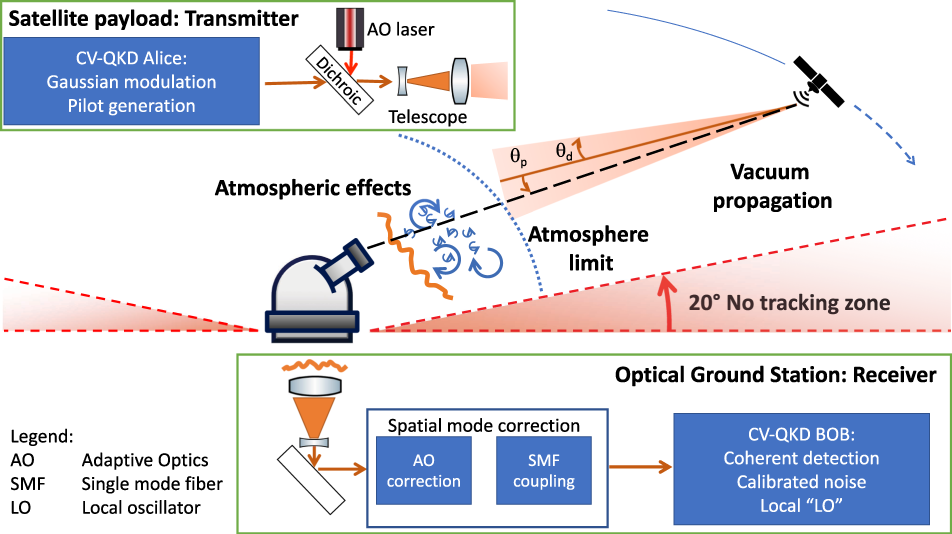The image depicts a detailed and colorful diagram of a satellite payload transmitter system, highlighting various technical components and their interactions. At the core of the diagram is a section labeled "Atmospheric Effects," illustrating the influence of atmospheric conditions on signal transmission. Key components include the ground station, satellite, and various elements like the CV, QKD, Alice, Gaussian Modulation, Pilot Generation, and multiple lasers, including the AO Laser. A telescope is depicted, accounting for spatial mode correction and atmospheric limits, with labels indicating a 20-degree no tracking zone.

A legend at the bottom clarifies abbreviations such as AO (Adaptive Optics), SMF (Single Mode Fiber), and LO (Local Oscillator), and details components such as the optical ground station receiver, coherent detection, and calibrated noise. The diagram shows signal pathways, marked by a dotted line illustrating vacuum propagation from the ground to the satellite. The chart uses various colors, including blues, pinks, and silver, for clarity.

This comprehensive illustration serves as a guide to understanding the complex interactions between satellite payload transmitters and ground stations, including how atmospheric effects, optical corrections, and signal propagation are managed within the system.